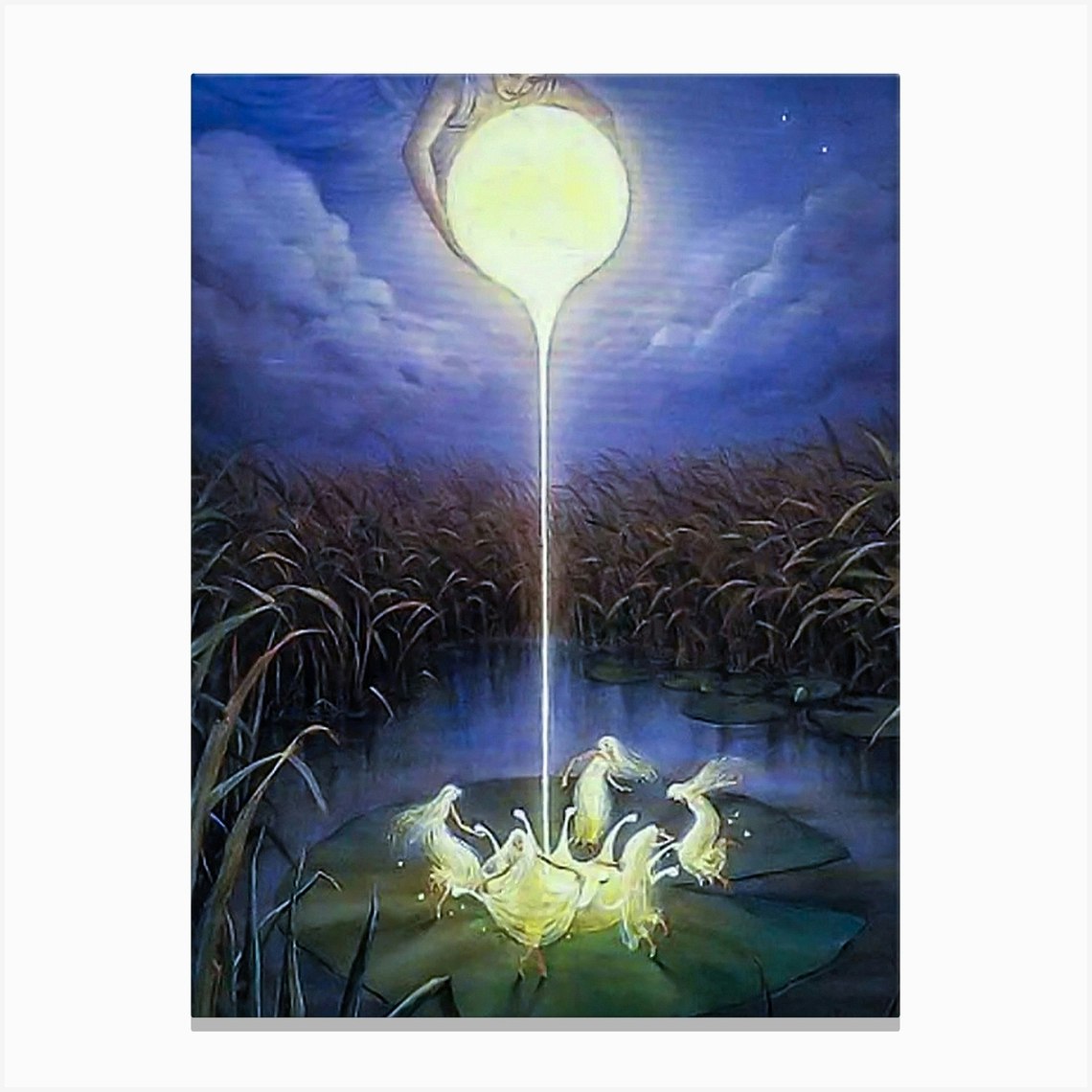In this enchanting digital drawing set in portrait mode, a celestial scene unfolds under a dark blue, cloud-filled night sky. At the top of the image, a luminous moon is being carefully poured out by a goddess, depicted in light yellow and gray tones. The goddess, wearing a white-strapped garment, has her face and arms visible as they delicately pour a mixture of white and gold from the moon. This ethereal liquid cascades downwards, illuminating the scene below. 

Beneath the celestial pouring, there is a canal-like space filled with tall, dark green, and dark purple grassy reeds, illuminated by the moonlight's glow. In the center of this magical pond, a larger lily pad takes prominence. Dancing atop this lily pad are five ghostly fairy-like figures, glowing in bright yellow. These ethereal fairies, adorned in long dresses and dancing shoes, seem almost to emerge from the splashes of the liquid moon. Their flowing long hair and the sense of movement they convey add to the whimsical, otherworldly atmosphere. The entire scene captures the essence of a nighttime fantasy, resembling a mystical illustration from a storybook page.